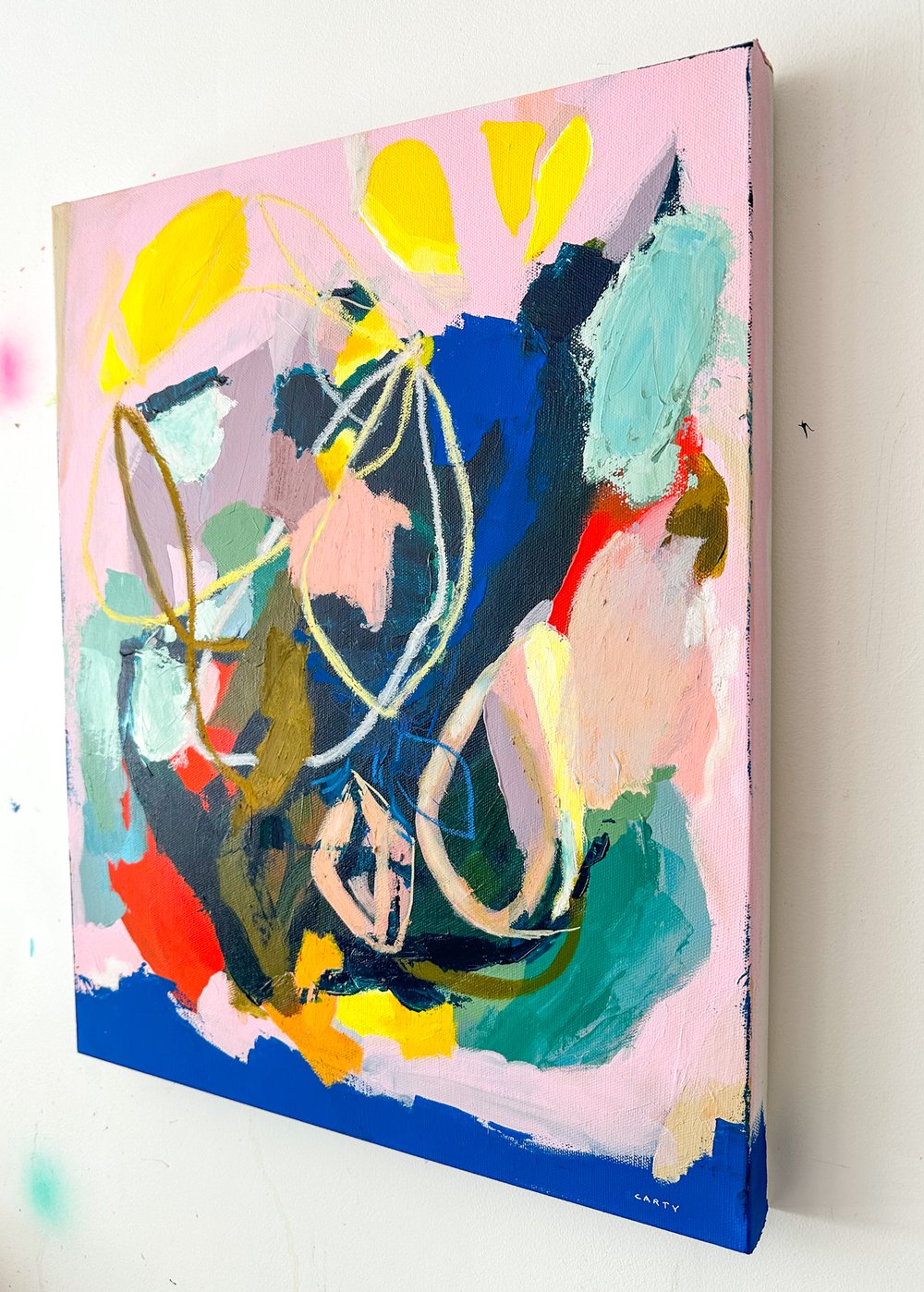The image captures a vibrant abstract canvas painting hung on a white wall, shot from a side view. The artwork is a pastiche of various vivid colors and patterns, prominently featuring shades of blue, pink, turquoise, yellow, orange, red, olive green, peach, and royal blue. The background is primarily light pink, extending almost the entire height of the painting, with an inch-high jagged blue line at the bottom. The composition includes a dynamic arrangement of circular patterns and flowing lines. In the bottom right corner, there is a white signature in all caps reading "CARTY," likely identifying the artist.